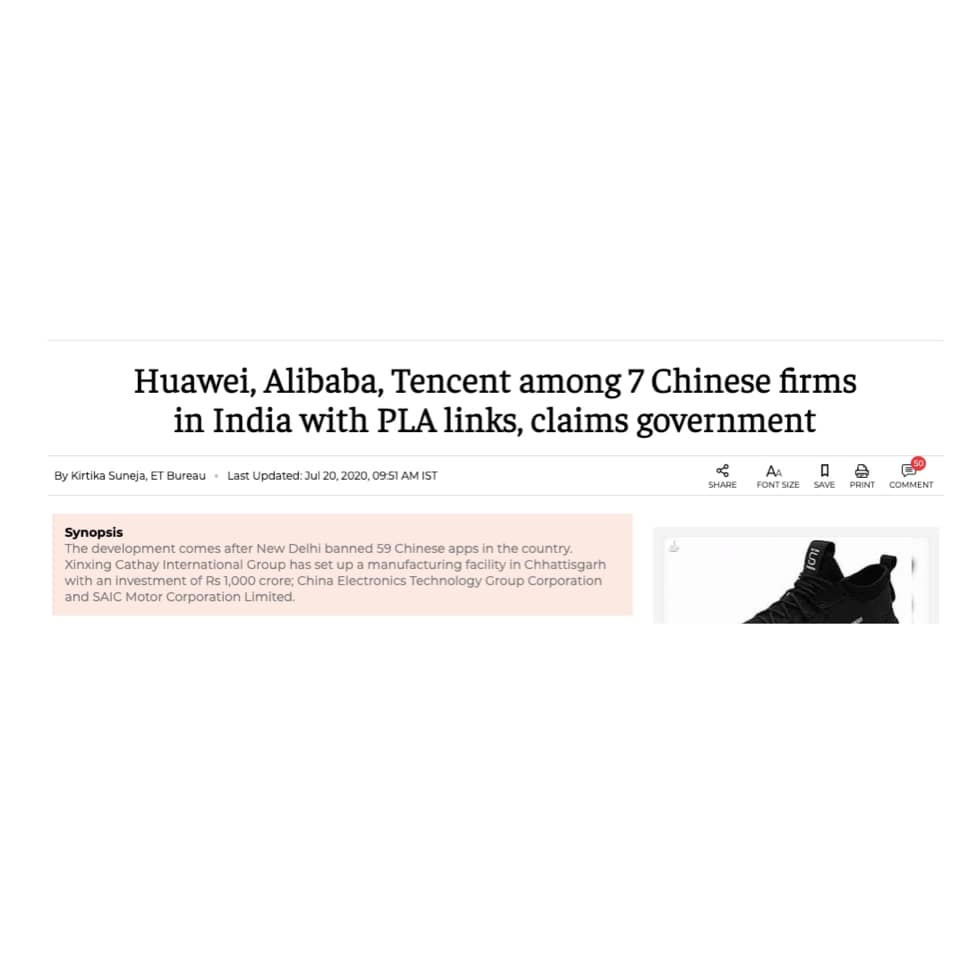The image appears to be a screenshot of an article with a white background. At the top, there's a grey line, followed by the article's title in black font: “Huawei, Alibaba, Tencent among seven Chinese firms in India with PLA links, claims government.” Below the title, another grey line separates it from the rest of the content. On the left side in very small black font is the byline: "By Kirtinka Sanijia, ET Bureau." Adjacent to it is a grey dash followed by "Last updated July 20th, 2020, 09:51 AM IST."

To the right, there are various icons and options. The share icon is accompanied by the text "Share," followed by font size adjustment options labeled "A," a "Save" button within a box, a "Print" button with a printer icon, and a "Comment" section shown as a square box with lines and a red circle containing a white number.

On the bottom left, there's a "Synopsis" section in black font with a pink background. This section starts with a grey font explaining the context: "The development comes after New Delhi banned 59 Chinese apps in the country. Xing Cathoway International Group has set up a manufacturing facility in Charistagra with an investment of RS1000 Crore. China Electronics Technology Group Corporation and SAIC Motor Corporation Limited..."

At the very bottom right corner, there is a grey outline of a black pair of running shoes.

This detailed caption encapsulates the visual layout and crucial textual elements found within the image.